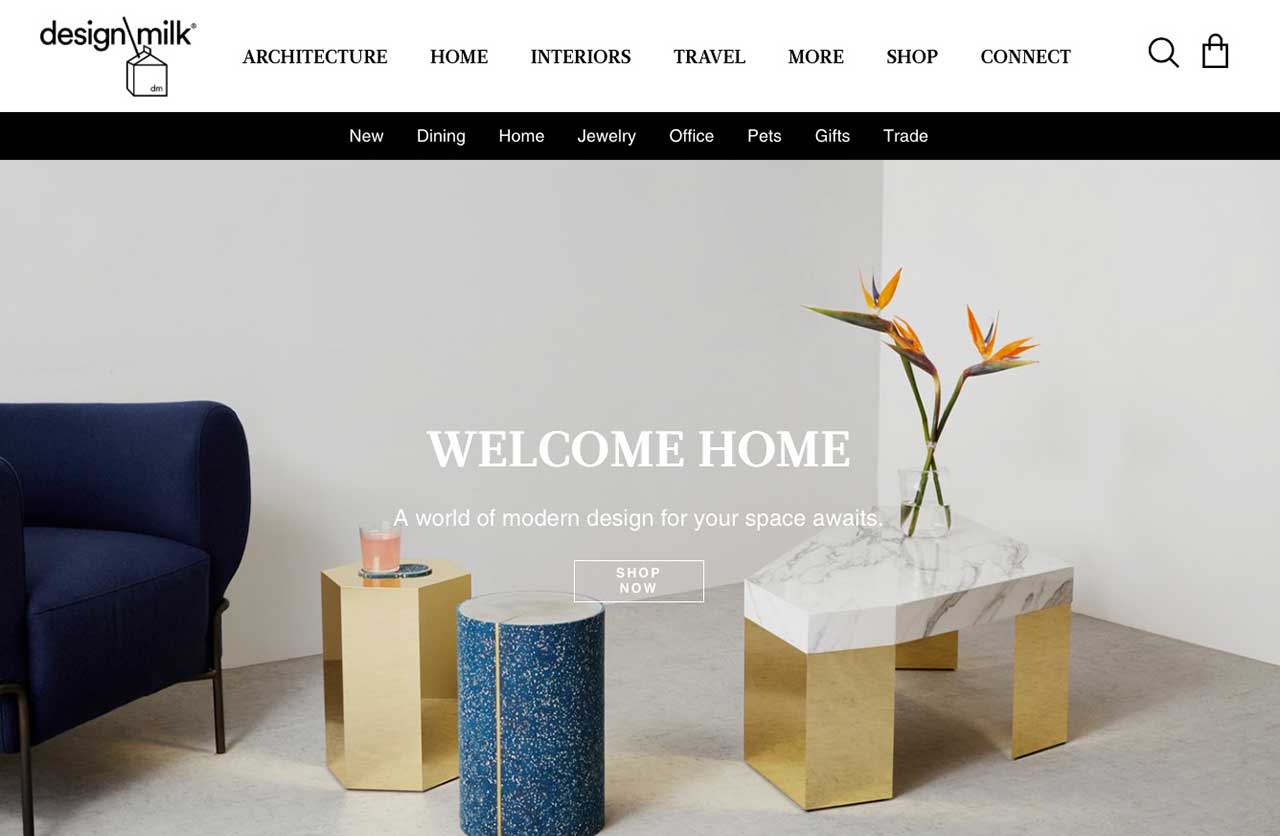This image from the website Design Milk features a meticulously organized landing page. At the very top, a white bar spans the width of the image. On the left side of the bar, "Design Milk" is written in black, with the text separated by a black and white milk carton icon featuring a black straw.

To the right of the logo, black text displays the website's main categories: "Architecture," "Home," "Interiors," "Travel," "More," "Shop," and "Connect." In the top right corner, black icons for search and shopping bag functionality are also visible.

Below the top bar, there is a black navigation strip listing categories such as "New," "Dining," "Home," "Jewelry," "Office," "Pets," "Gifts," and "Trade," all written in white text.

The main focus of the image is a showroom display area. On the left side, a blue chair with black legs catches the eye. Centrally positioned are two tables; one has a gold finish and the other is a bluish round table. Additionally, a white table in the center is adorned with a bouquet of flowers, adding a touch of nature to the sophisticated setting.